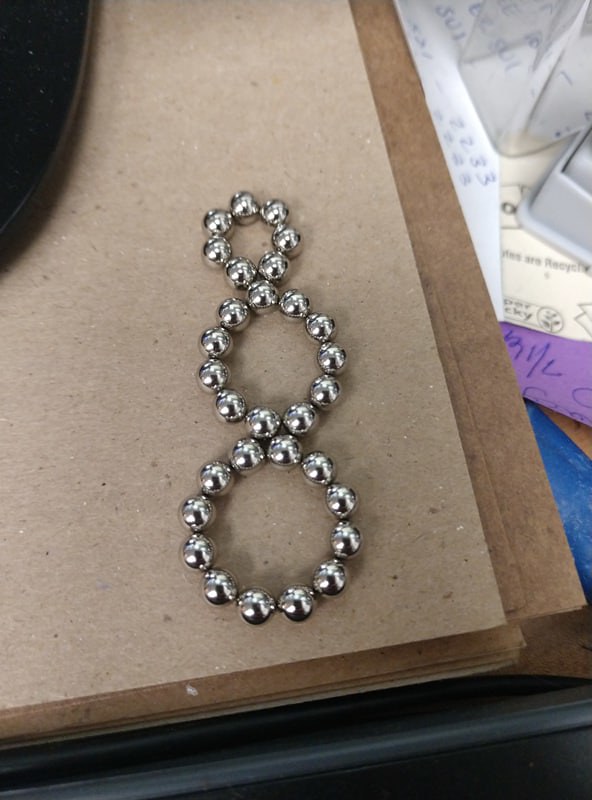The color photograph captures a piece of jewelry comprising three interlinked hoops made of shiny silver metal beads or small bell-like elements. The hoops, arranged in ascending order of size from top to bottom, form what looks like a fluid chain with the largest circle at the bottom and progressively smaller circles towards the top. The smallest hoop is topped with seven tiny beads that resemble miniature bells often found on pet collars. These intricate metal rings are set against a brown, paper-textured background, which may be thin wooden boards or cardboard slabs. To the right of this elegant piece, there is a cluttered stack of various papers, notepads, and printouts, though their content remains undecipherable. This chaotic paper arrangement adds a contrasting element to the neatly stacked brown backdrop, which some might perceive as a dark wooden shelf or table.